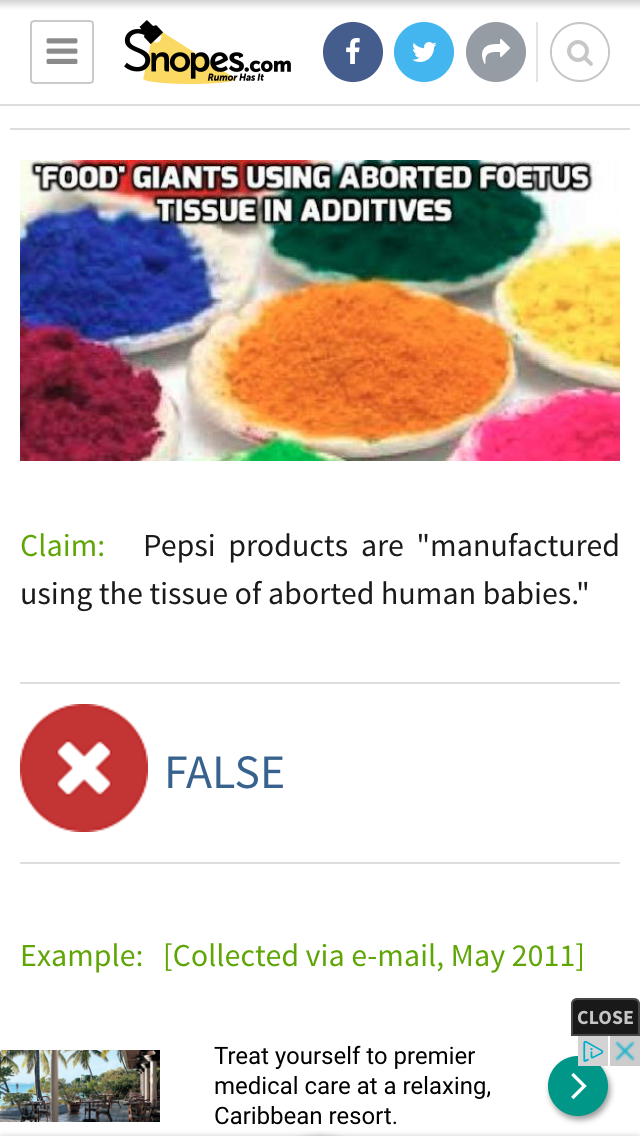The image is a tall, rectangular screenshot of a Snopes.com webpage, with a white background and a thin gray line at the top. Underneath, the Snopes logo, depicting a lamp shining a yellow light, is displayed alongside the tagline "rumor has it." To the right of the logo are icons for Facebook, Twitter, and a possible share button, as well as a magnifying glass for search functionality. 

Below this header, there is a wide rectangular photograph showcasing an array of small white circular platters, each filled with a different color powder—orange, dark green, yellow, blue, red, and pink. Superimposed over the photograph in bold white font with black borders is the text: "Food giants using aborted foetus tissue in additives." 

Beneath this, the word "Claim" appears in green, followed by text in black that reads: "Pepsi products are manufactured using the tissue of aborted human babies." A prominent red circle with an "X" through it, labeled "False," indicates the claim's veracity. Below this section, it notes "example collected via email May 2011," and at the bottom of the screenshot, there's an advertisement.